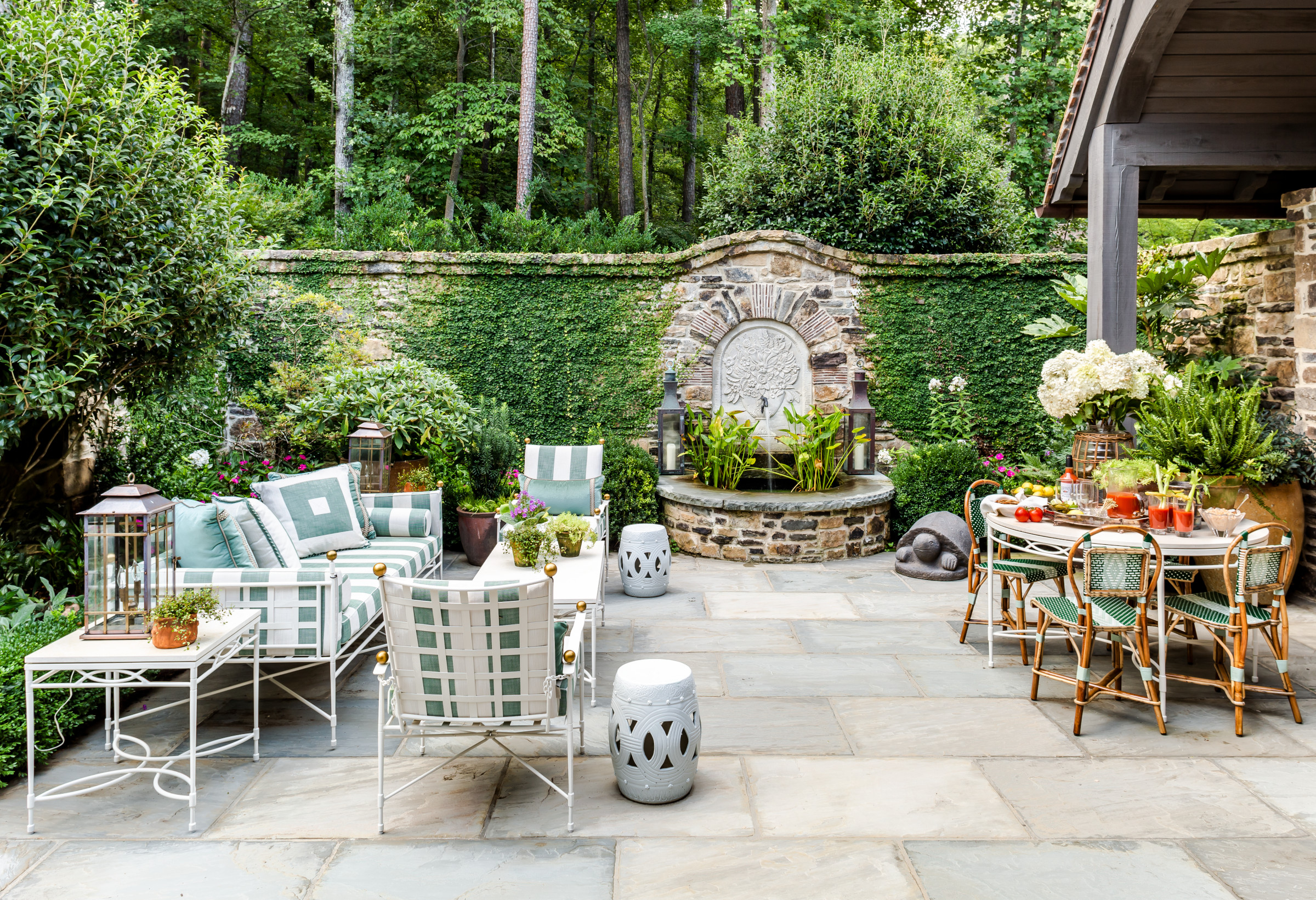This image captures a beautifully landscaped outdoor patio, likely part of a home's backyard. The area features a spacious, rectangular brick-tiled floor with light gray and white hues. A sturdy stone wall, covered in verdant ivy, forms the backdrop, adding texture and a touch of antiquity. A charming fountain, set into the wall, features water trickling from a quaint faucet into a basin filled with lush green plants. Tall, leafy trees frame the scene, providing a sense of seclusion and natural beauty.

To the right of the image, there is a white wicker table surrounded by bamboo-like wooden chairs, adorned with tomato juice glasses garnished with celery stalks, along with an assortment of fresh fruit. On the left, a cozy seating arrangement includes white metal-framed couches and chairs, cushioned with attractive green and white striped fabric, evoking a relaxed yet sophisticated ambiance. Near this seating area, a smaller table with a lamp and several decorative plants enhances the inviting atmosphere.

Additional details include a stone turtle ornament perched in one corner, a candle holder on a side table, and moss spotting the stone wall, contributing to the lush, vibrant aesthetic of this tranquil patio setting.